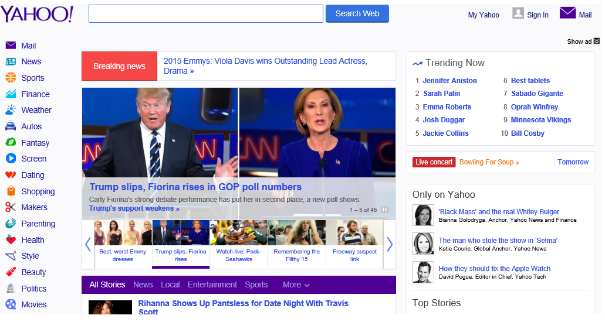The image is a screenshot of the Yahoo homepage. Prominently displayed in the top left corner is the recognizable Yahoo logo. On the left side of the page, there is a vertical menu list that spans the entire length of the left-hand side. The central portion of the screen highlights breaking news, featuring a photograph of Donald Trump alongside another image of a woman. The headline associated with Trump reads "Trump slips, Fiorina rises in GOP poll numbers." Next to this, a headline highlights "2015 Emmys: Viola Davis wins Outstanding Lead Actress in a Drama." Below these main headlines, a menu scroll bar is visible. On the right-hand side of the page, there are sections labeled "Trending News" and "Only on Yahoo."